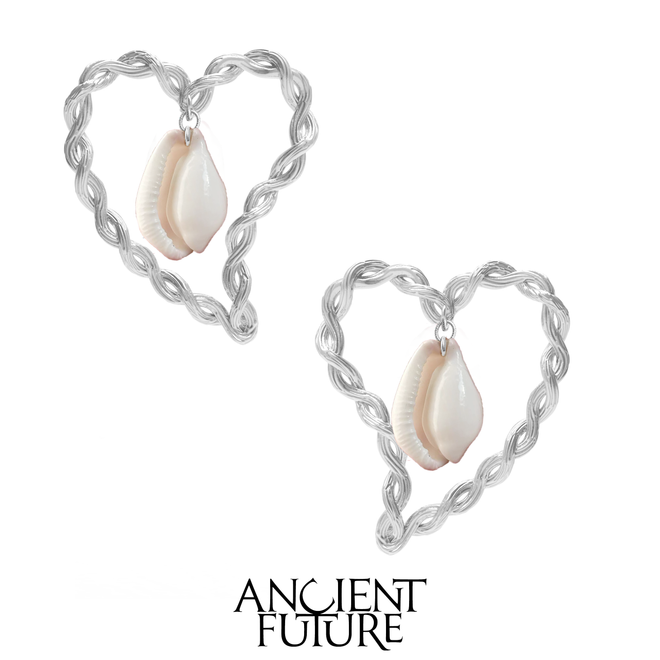This product photograph features a pair of intricately designed jewelry items set against a solid white background, creating the effect that the pieces are floating in an empty void. The image includes two heart-shaped items, which could be pendants or earrings, both made from twisted silver metal that subtly resembles a DNA helix before forming into a slightly skewed heart shape. Each heart is adorned at the center with a small hoop, from which a miniature, delicate seashell dangles. The seashells are pale pink and exquisitely detailed. The overall shape of the photograph is rectangular, with a duo of black text lines at the bottom reading "Ancient" and "Future," where the 'C' in "Ancient" is notably tilted at an angle. These stylish pieces are likely crafted by a jeweler represented by the name "Ancient Future."